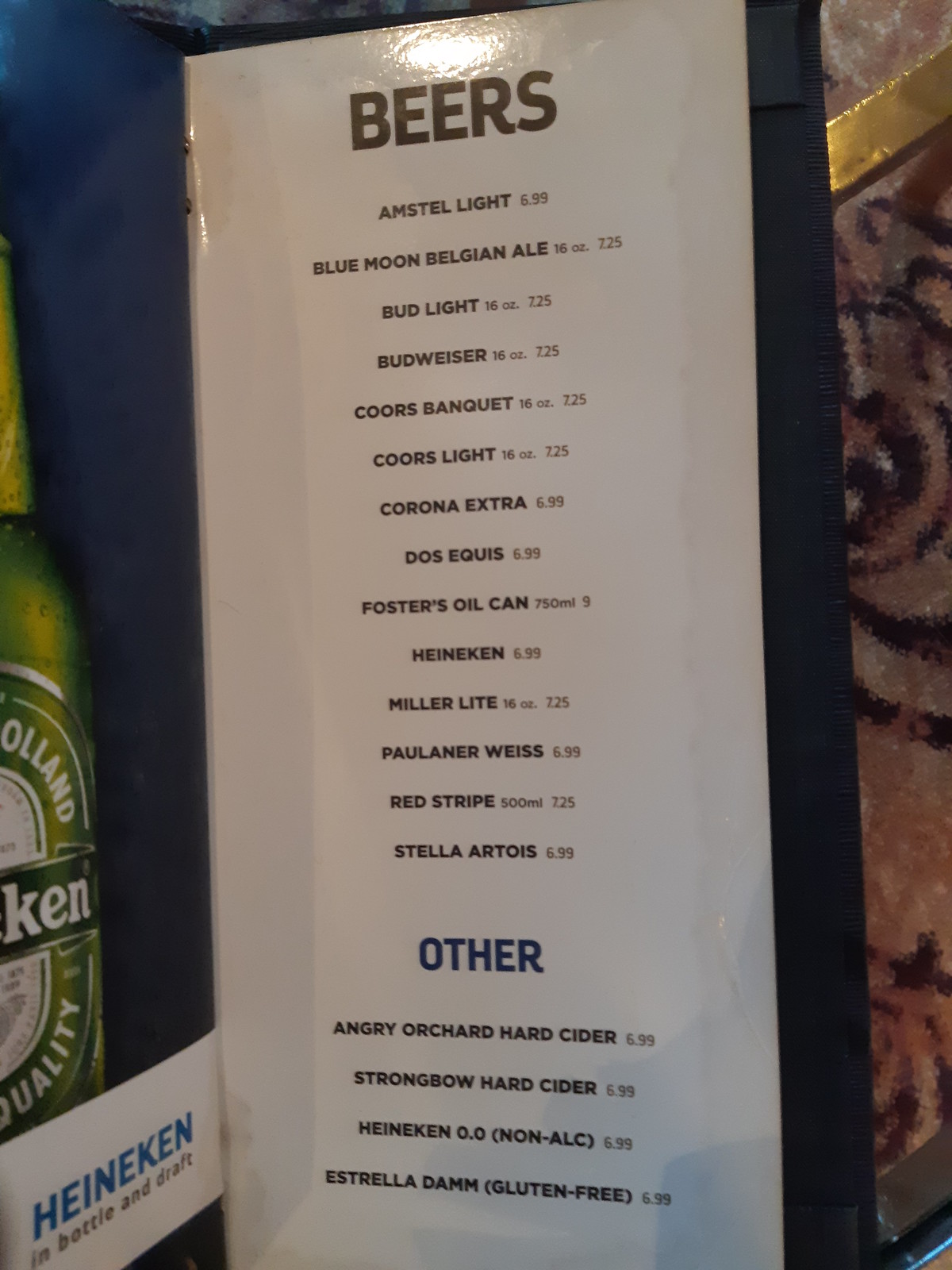A meticulously crafted bar menu set against a distinctive wooden surface with swirling dark patterns. The menu itself is stark white, providing a clear contrast to its rich background. On the left side, there's a vivid image of a Heineken can, underscored by the name "Heineken" in blue lettering. The menu is titled "Beer" and details an extensive list of beer options along with their prices:

- **Amstel Light**: $8.95
- **Blue Moon Belgian Ale**: $7.25
- **Bud Light (16 oz)**: $7.25
- **Budweiser (16 oz)**: $7.25
- **Coors Banquet (16 oz)**: $7.25
- **Coors Light (16 oz)**: $7.25
- **Corona Extra**: $6.99
- **Dilsake**: $6.99
- **Foster's Oil Can (750 ml)**: $9.00
- **Heineken**: $6.99
- **Miller Lite (16 oz)**: $7.25
- **Paulaner Weissbier**: $6.99
- **Red Stripe (500 ml)**: $7.25
- **Stella Artois**: $6.99

Beneath the "Other" category in blue letters:

- **Angry Orchard Hard Cider**: $6.99
- **Strongbow Hard Cider**: $6.99
- **Heineken (Non-Alcoholic)**: $0.00 (marked $6.99)
- **Estrella Damm (Gluten Free)**: $6.99

This detailed menu offers a wide array of choices for beer aficionados, meticulously listing popular brands and their corresponding prices.